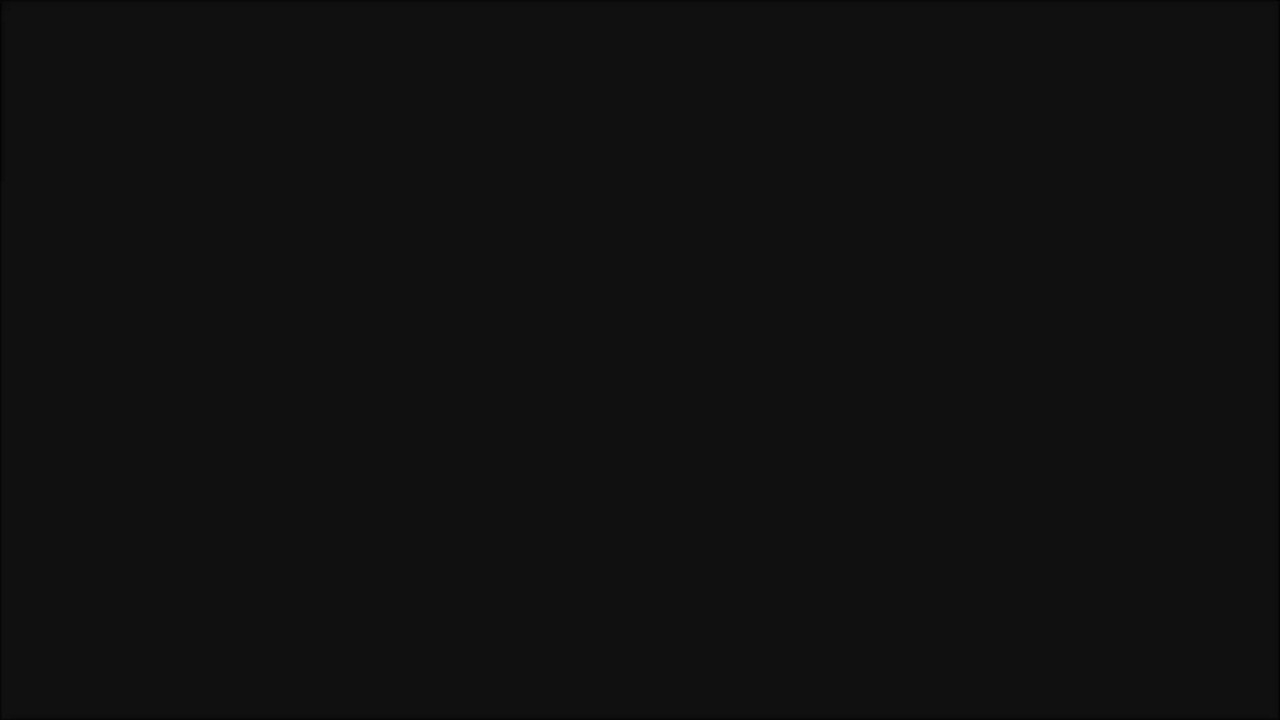A screenshot displayed in the image is entirely blank, showcasing a completely black screen. There are no discernible objects, text, or subtle details visible within the image. The absence of any visual elements suggests a possible technical fault. The background remains uniformly black, lacking any stylistic elements or features. This image was expected to display a website, but instead, it is just an empty black square, indicating an issue that likely requires further technical investigation.